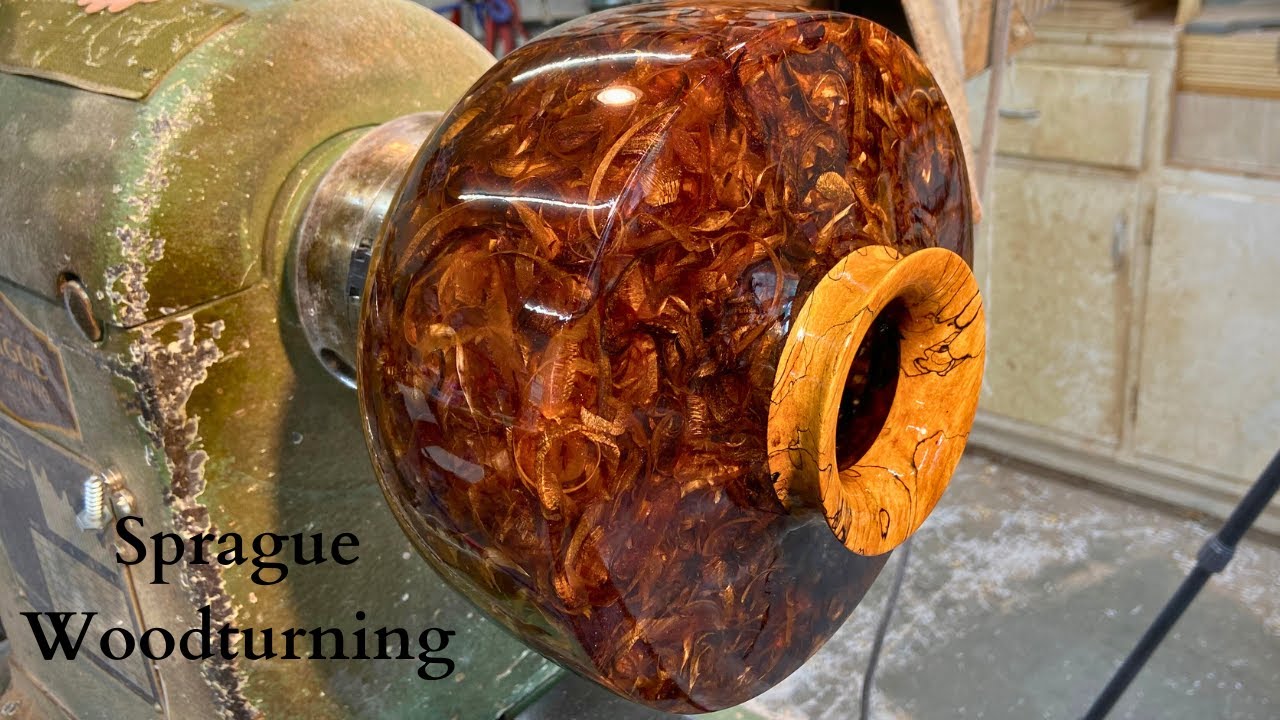In a spacious warehouse adorned with white shelving units, an industrial machine dominates the left side of the image, standing on a light gray floor. The machine itself is a noticeable combination of gray and light yellow, weathered with signs of rust and wear. Affixed to this lathe is an intricate piece of craftsmanship: a gleaming, shimmering brown vase. The vase, likely a product of epoxy or resin casting intermingled with woodwork, exhibits a rich light brown hue with a glittery, almost suspended-in-water effect, suggesting a highly polished finish. The top of the vase features a golden-yellow rim, accentuating its ornate design. This vessel, possibly filled with wood shavings, is an advertisement piece for Sprague Woodturning, hinting at the company's focus on turning wood into exquisite objects.